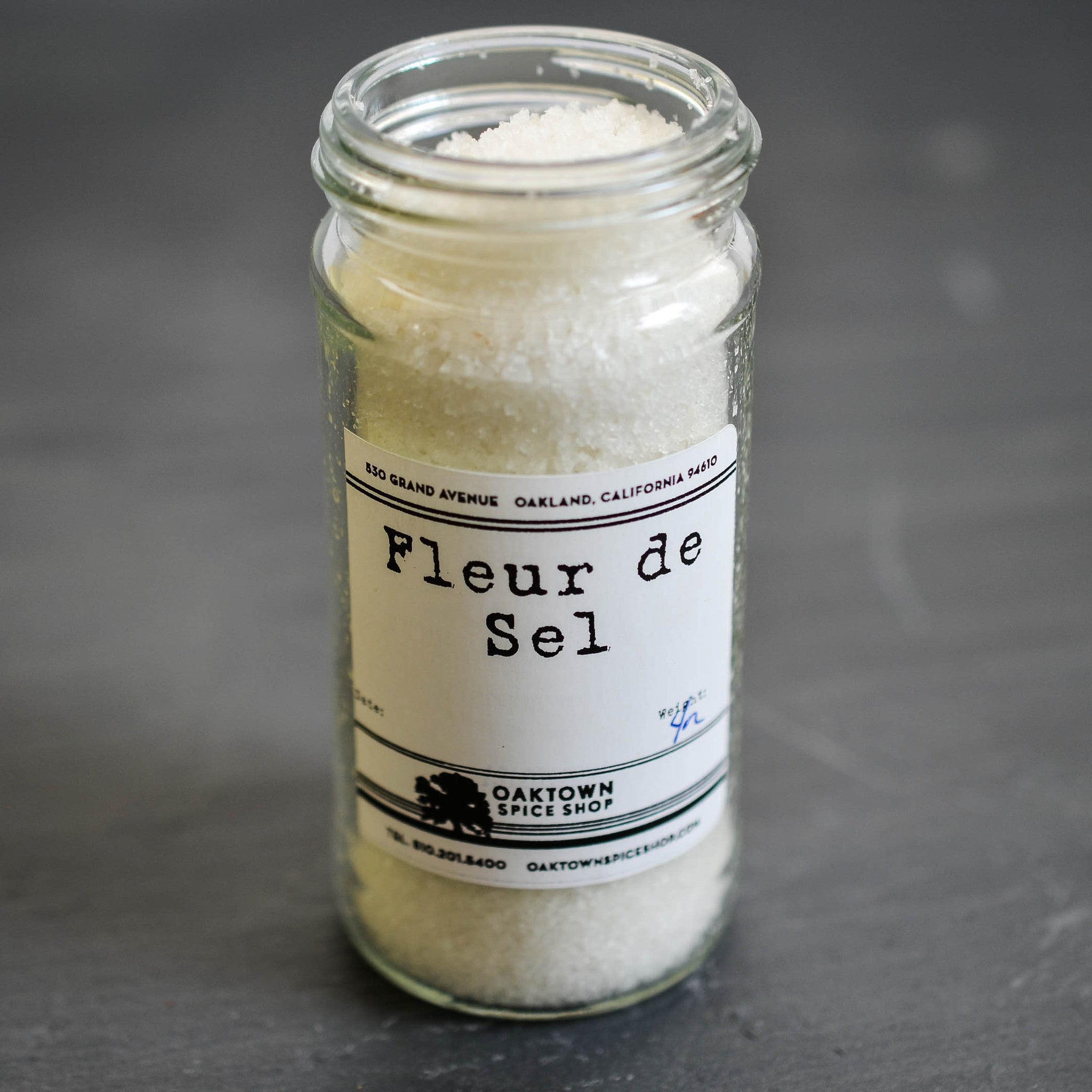The image depicts a high-quality, clear glass salt dispenser without a lid, filled with a white substance presumed to be salt or Fleur de Sel. The primary focus is on this jar, which takes up the majority of the image, set against a blurred dark or gray surface that obscures specific details of the background. The jar features a black and white label stating the address "830 Grand Avenue, Oakland, California, 94610" and identifies the contents as "Fleur de Sel" from the "Oaktown Spice Shop". The label also includes an indistinct telephone number and website, with a logo of a tree overlaid by horizontal lines. The overall image has a soft focus, particularly blurring out the surrounding area, which might be a table or floor.